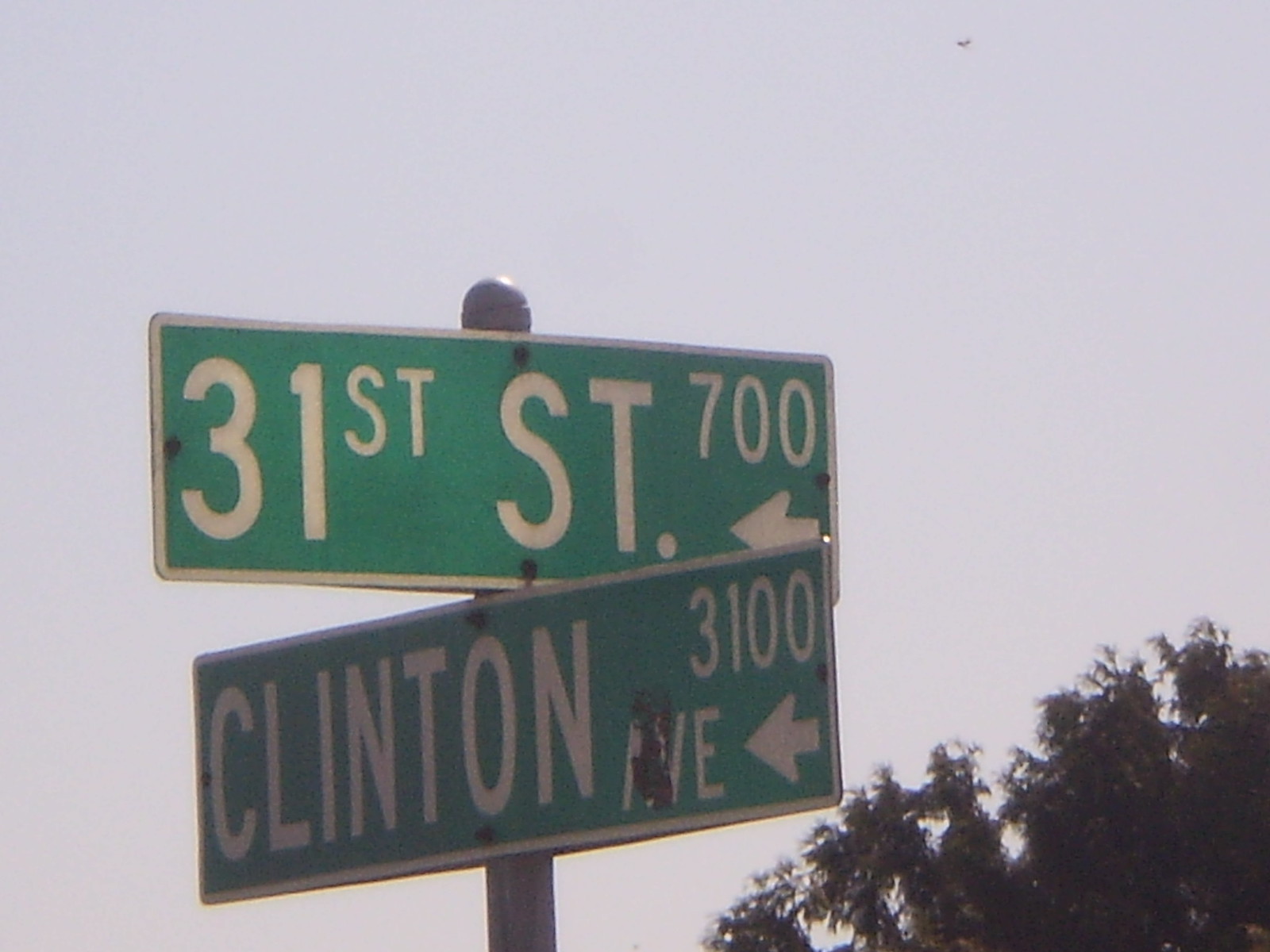In this outdoor photograph, two street signs prominently stand against a backdrop of a grayish-blue sky, which appears overcast without visible clouds, presenting a muted atmosphere devoid of sunshine. The street signs are mounted on a robust, gray metal cylindrical post, capped with a rounded top. In the bottom right corner of the image, dark green foliage from a tree adds a touch of nature to the urban scene. The top street sign is green with a white border and white text, reading "31st St." It features the number "700" with a white arrow pointing left. Below it, another green sign with similar styling bears the name "Clinton Ave" (abbreviated as "AVE"), along with the number "3100" and another left-pointing arrow.